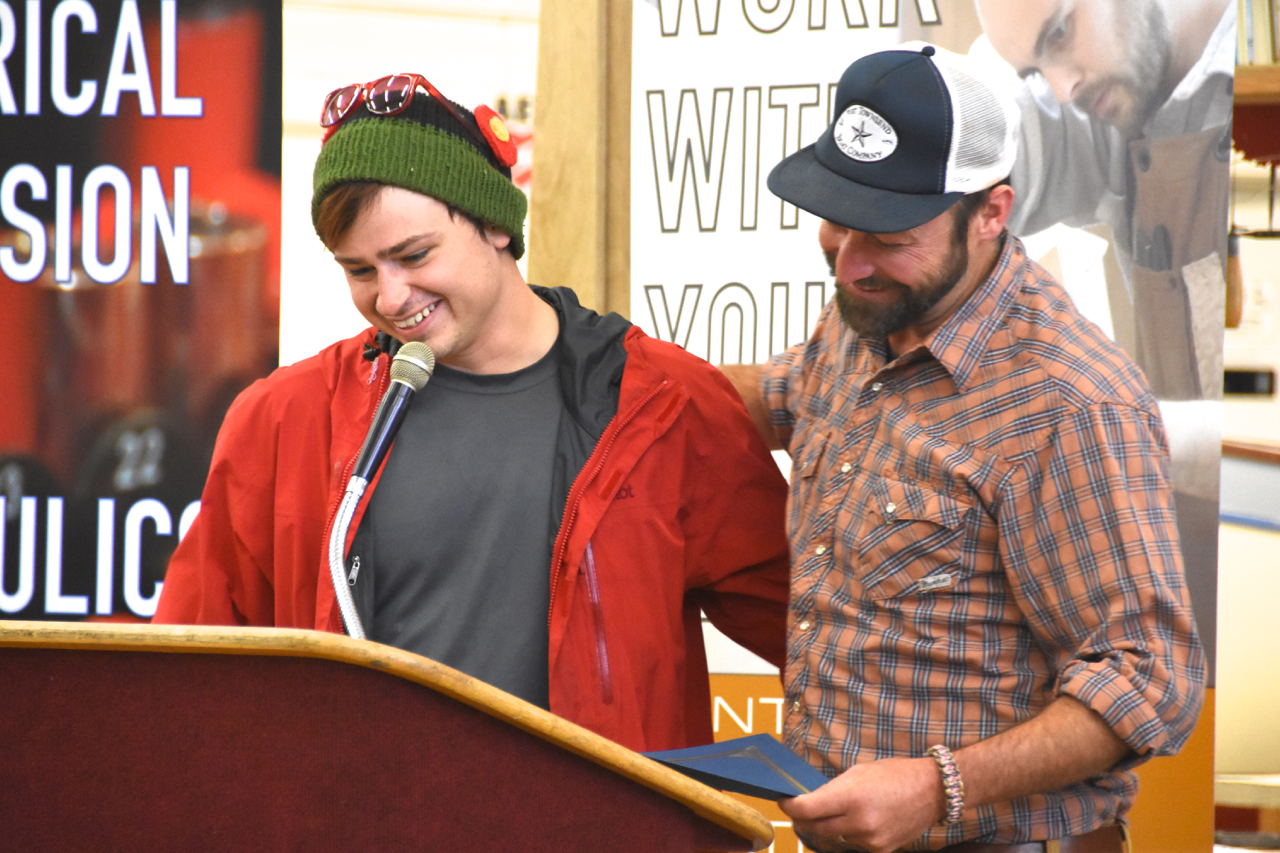In this vibrant and heartwarming image, two men stand behind a light wood-framed podium, clearly ready to address an audience. Both are smiling broadly, their joy palpable. The man on the left, who appears to be in his 20s, wears a black beanie with a green rim and red sunglasses perched on top of his head. He is dressed in a red jacket over a gray shirt, and his gaze is directed warmly down at the podium. The man on the right, exuding a casual yet friendly demeanor, wears a navy blue and white baseball cap, a plaid shirt with rolled-up sleeves, and a bracelet on his left wrist. He has his left arm around the younger man and holds a blue pamphlet in his left hand, smiling cheerfully down at the podium. Surrounding them is an evident backdrop, featuring large, partially visible banners and signs with text. The banners add a vibrant splash of red and white to the scene, hinting at some form of advertisement. Both men share a moment of camaraderie and anticipation, likely preparing to make a speech, as emphasized by the microphone emerging from the podium.